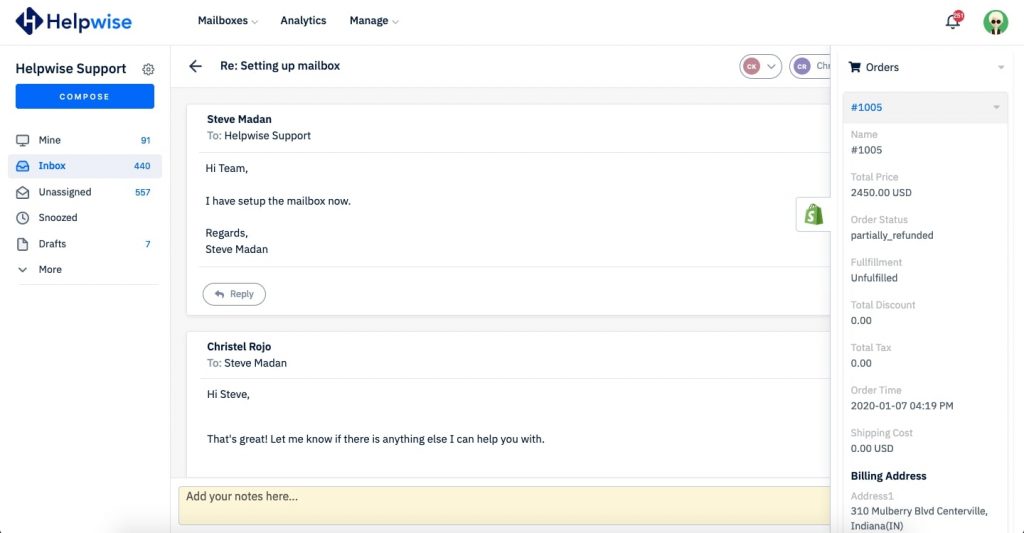This image is a screenshot of a Helpwise email platform interface, presented in a landscape format. The background seamlessly blends into the white interface of the screen, making it appear continuous.

In the upper left-hand corner, the Helpwise company logo is displayed. The logo consists of a blue square with a stylized, zigzagged "H." To the right of the logo, three tab options are visible: "Mailboxes," "Analytics," and "Manage." A thin horizontal line spans the width of the screen beneath these tabs.

On the left side beneath this line, a section titled "Helpwise Support" is visible. A prominent blue button labeled "Compose" suggests functionality to draft new messages. The sidebar lists various email categories including "Mine," "Inbox," "Unassigned," "Snooze," and "Drafts."

The main window displays an email conversation between Steve Madden and Helpwise Support. Steve Madden's message reads: "Hi team, I have set up the mailbox now. Regards, Steve Madden." Following this, Crystal Rojo from Helpwise Support replies: "Hi Steve, that's great. Let me know if there's anything else I can help you with."

On the right-hand side of the interface, a drop-down menu is present with options related to "Orders" and a "Billing Address," indicating additional functionality or account management features. The mention of Centerville, Indiana, suggests the location context of the correspondence.

Overall, the interface portrayed is that of a company’s internal email communication platform, designed for customer support and administrative functionalities.